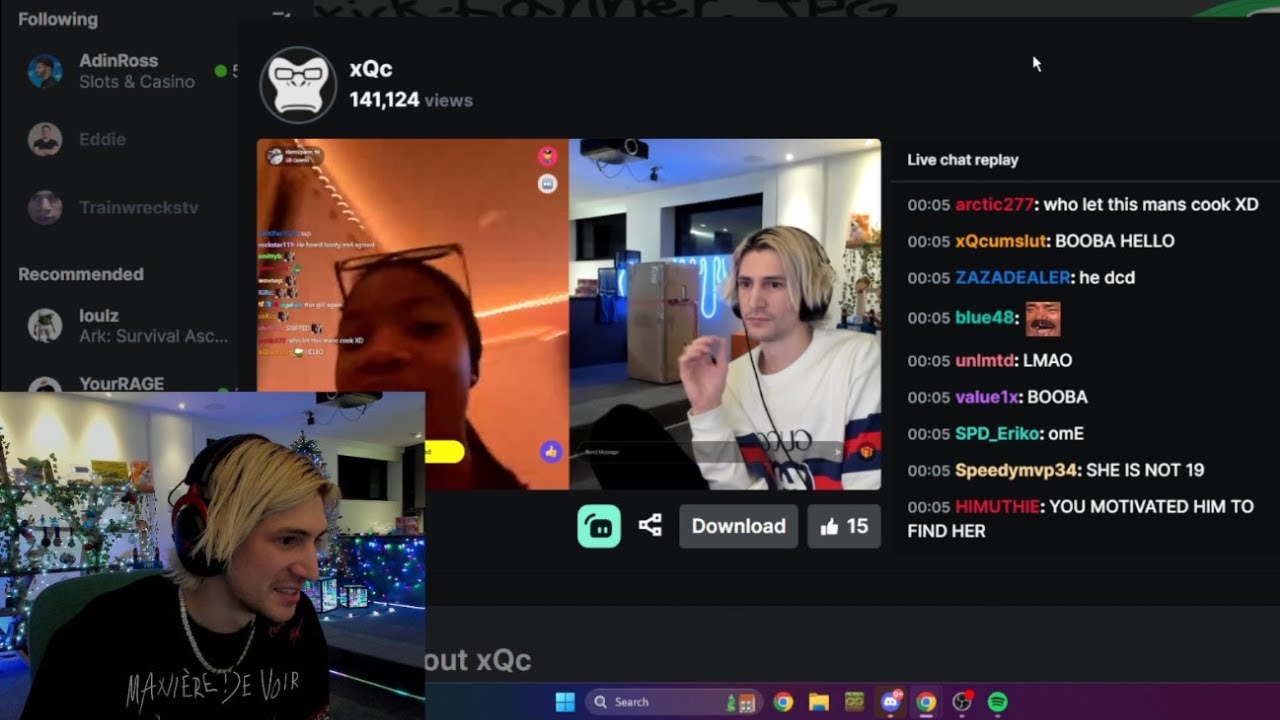In this lively streaming session, three individuals are engaged in a dynamic broadcast. On the bottom left, a blond-haired man wearing headphones and a necklace is visibly present. In another frame, the same man appears again, this time in white long sleeves and still sporting his headphones. Additionally, a woman with glasses contributes to the trio of streamers.

The screen is peppered with various names and tags, including Aden Ross, Sloth, Casino, Eddie, Trainwreck STV, Louise, Ark Survival, Your Rage, and XQC. The stream has garnered significant attention, boasting 141,000 views and 824 active participants in the Live Chat Replay, indicating a vibrant and highly interactive audience.